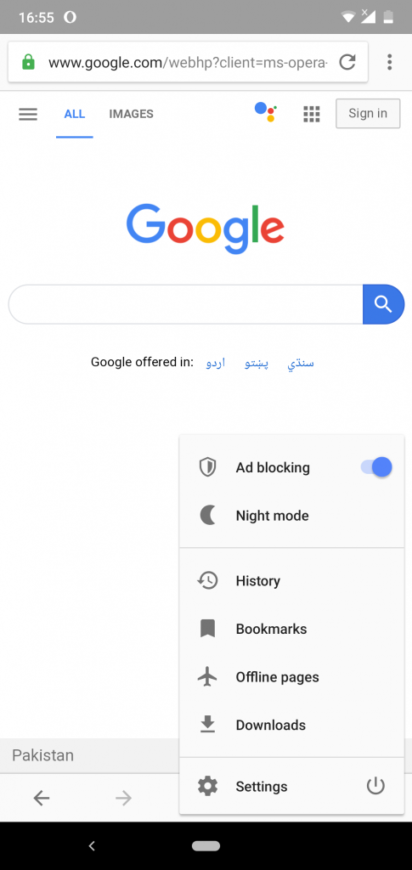A screenshot taken at 16:55 shows the familiar layout of a Google search page within a web browser. In the top left corner, the letter "O" is displayed, while the top right corner features a Wi-Fi symbol, a data signal icon, and a battery indicator. The top section of the browser has a gray background. Just below this is the URL bar, highlighted by a green padlock and the URL "www.google.com/webhp?client=ms-opera," accompanied by refresh and options icons (three dots). 

Directly below the URL bar, the screen displays navigation options including an underlined "All", "Images", and the Google Apps grid icon, followed by a "Sign in" button. The prominent Google logo, spelled "G-O-O-G-L-E" in the company's signature blue, red, yellow, and green colors, is centrally located above a search bar. The search bar features a white search icon on a blue background.

Underneath the search bar, Google offers its services in three foreign languages. A pop-up menu with various options like ad blocking (with a blue toggle), night mode, history, bookmarks, offline pages, downloads, settings, and a power button appears. 

To the left side of this panel, "Pakistan" is denoted below a horizontal line, indicating the user's location or preference. The bottom of the screen has visible back and forward arrows. The footer section is black and contains a small white bar and another back arrow icon.